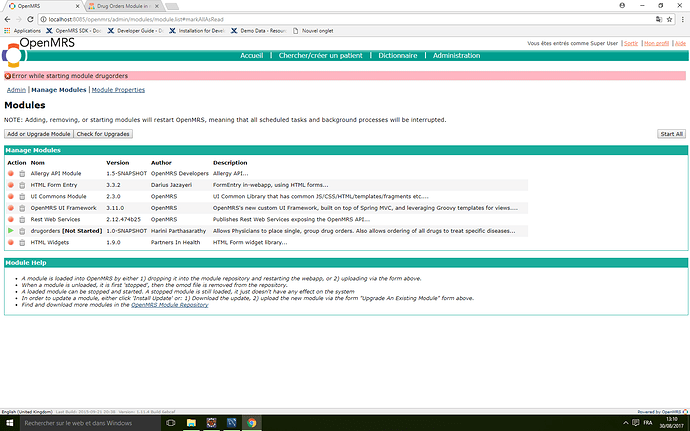A small, zoomed-in image displays a web browser window with several open tabs and a visible search bar. Below the search bar, a bookmark bar showcases six different bookmarks. Intricate details include an "OpenMRS" section featuring a circular logo with distinct color segments: red at the top, blue on the left, yellow at the bottom, and teal on the right, with the teal section extending across the image. Interactive elements labeled "Account," "Dictionary," and "Administration" are visible. A prominent pink area indicates an error message stating, "Error while starting module: Drug Orders." Beneath this message are options for "Admin," "Manage Module," and "Module Properties," along with a note that adding, removing, or starting the module will restart OpenMRS.